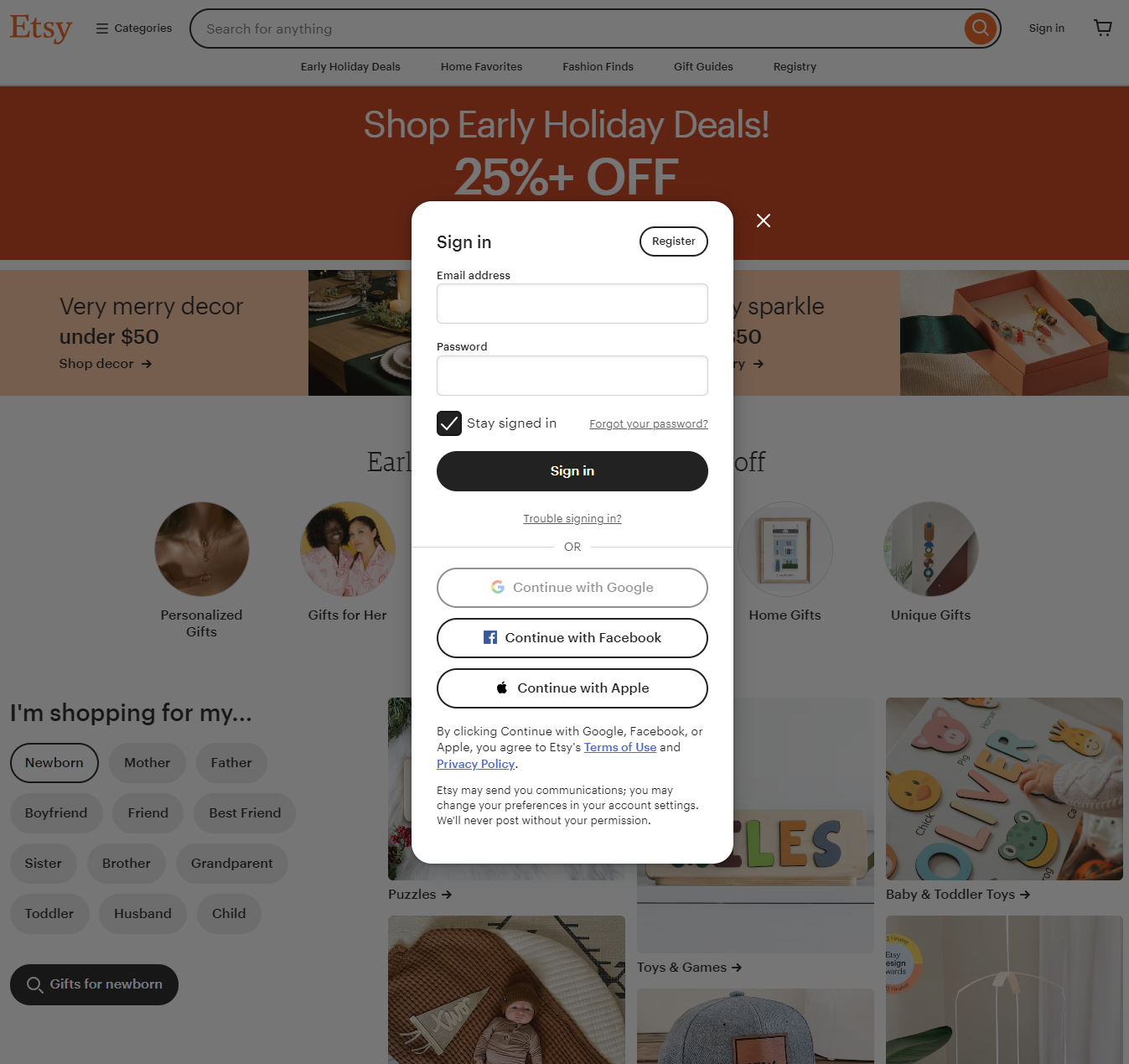The image displays a faded Etsy webpage with a central dialog box prompting the user to sign in. The dialog box is titled "Sign In" in bold, black lettering and provides options to either sign in or register if the user does not have an account. Below, fields for entering an email address and password are present, accompanied by a check mark box labeled "Stay signed in," which is currently checked. Alternative sign-in options include continuing with Google, Facebook, or Apple. A disclaimer states that continuing signifies agreement to Etsy’s terms.

In the background, partially obscured by the dialog box, the Etsy website header is visible with "Etsy" prominently displayed in orange. The top navigation bar features a category section, a search button in the center, and options to sign in or view the shopping cart on the right. Below, an orange banner announces "Early Holiday Deals" and a prominent button invites users to explore "Home Favorites," "Fashion Finds," "Gift Guides," and "Registry" categories. The promotional section boasts a "Shop Early Holiday Deals: 25% Off Plus" offer and includes an orange banner stating "Very Merry Decor Under $50," with a clickable button to shop decor. 

The screen also shows a shadow box featuring some jewelry, although partially hidden by the dialog box, with text indicating "Sparkle" or a similar heading. Below the banner, a selection of themed gift sections is visible, such as "Personalized Gifts," "Gifts for Her," and "Home Gifts." 

At the bottom left of the webpage, a section titled "I'm Shopping For" offers clickable choices with corresponding images, including "Newborn," "Mother," and "Father." The user selects "Newborn," revealing further options like "Gifts for a Newborn," "Baby and Toddler Toys," and a few other categories. Each category is accompanied by representative images to guide the shopper.